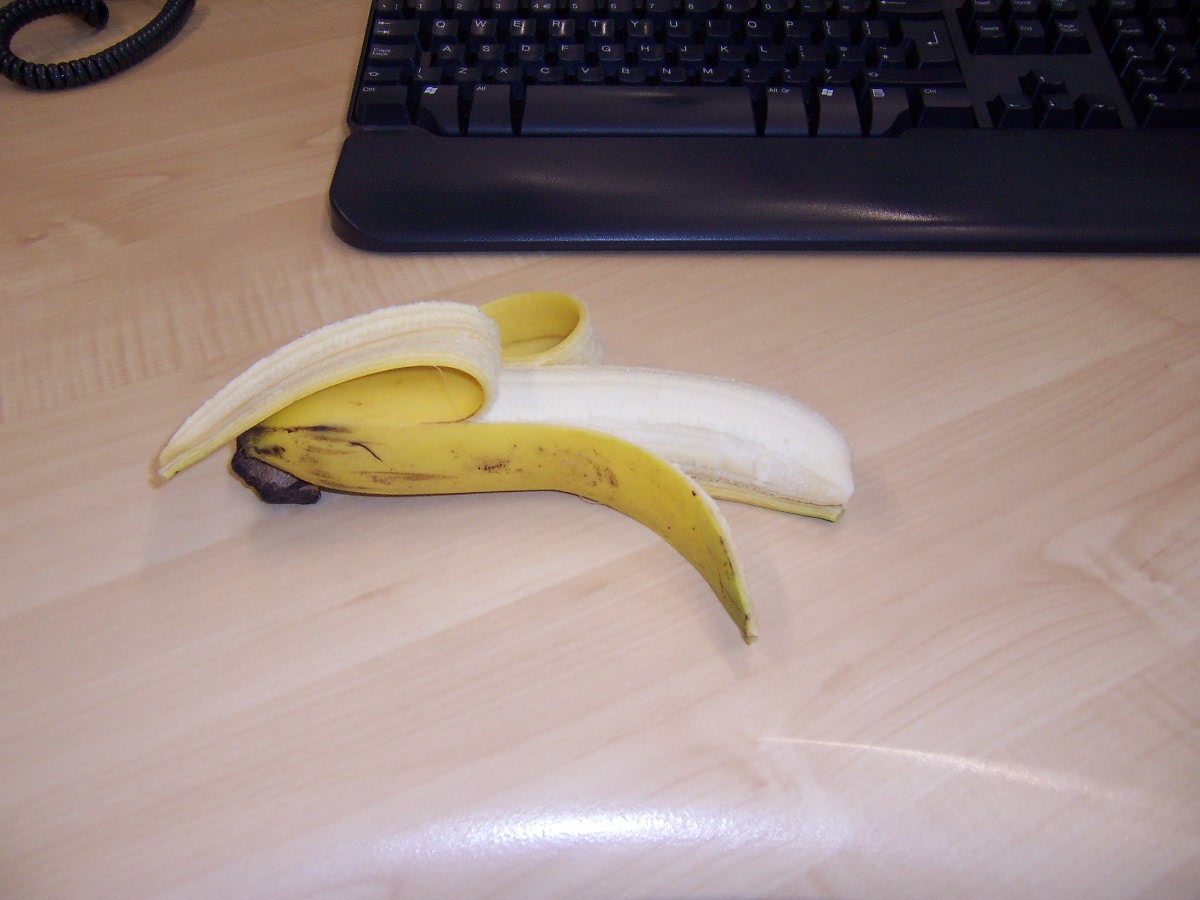A single, partially peeled banana is prominently displayed in the center of the image. The peel is divided into four sections. One section is peeled about two-thirds of the way down and folded over, another is peeled halfway and folded back, the third section is peeled slightly less and partially pulled open, while the fourth remains unpeeled and lies flat beneath the banana. The banana itself shows a few black spots, mostly at the base, and small marks on the peel, but the fruit appears unmarked. The scene is set on a light wood table. In the background, a black keyboard spans the upper part of the image, extending to the right where it is cut off around the number pad. On the left side, a spiral phone cord ascends and is truncated at the image’s edge. There is a noticeable glare in the bottom right corner, and a faint reflection at the top, obscuring parts of the keyboard up to the F12 keys.